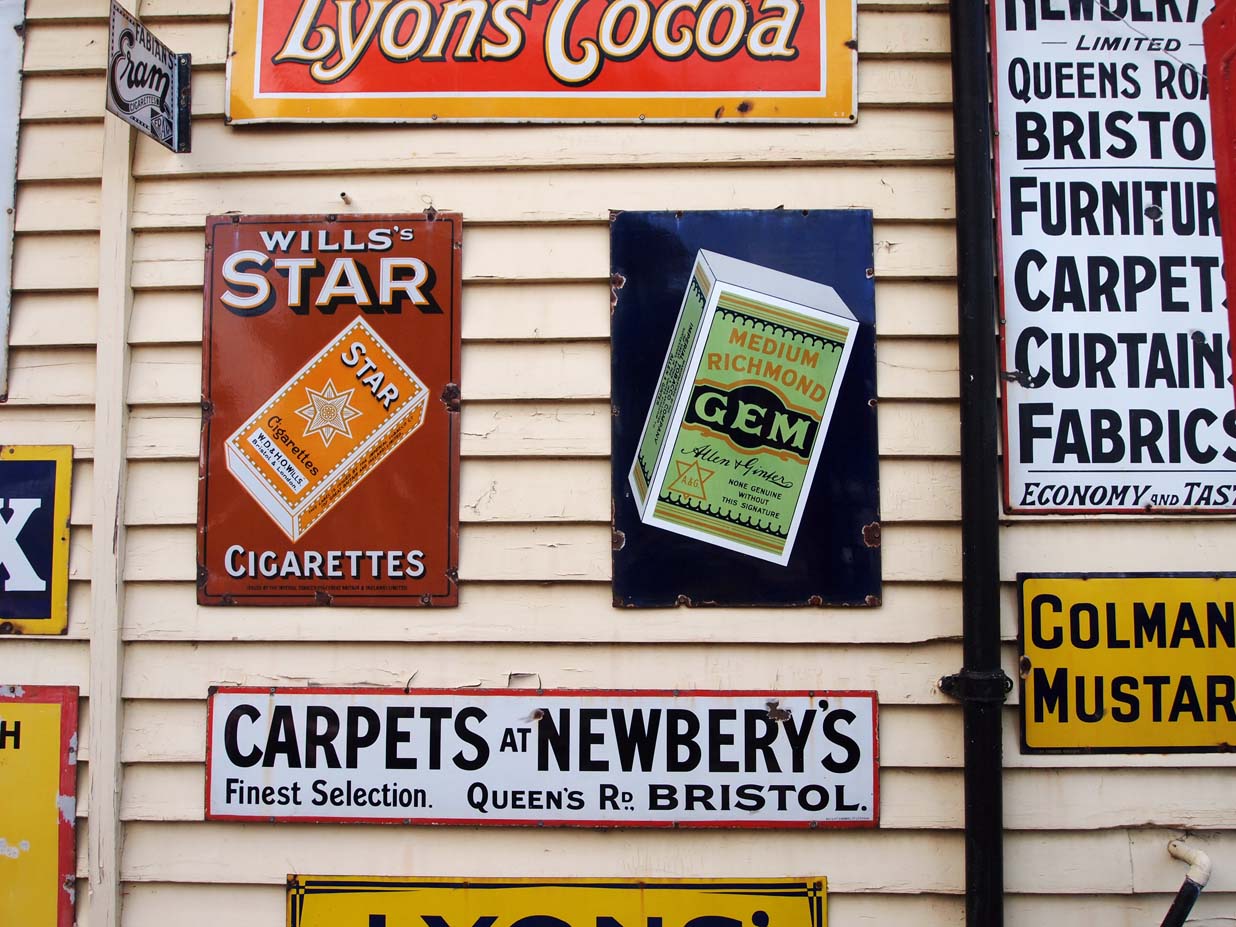This photo showcases a collection of vintage metal signs affixed to a light brownish-green, slotted siding of a building. At the top, a vibrant orange-red sign reads "Lion's Cocoa." Directly below, a vertically positioned sign with a brown background features an image of an orange cigarette box and the text "Willis Star Cigarettes." To the right of it, another vertical sign with a blue background presents a green box labeled "Medium Richmond Gem." Below these, a horizontal white sign outlined in red advertises "Carpets at Newberry's Finest Selection, Queen's Road, Bristol." The image also includes various other signs that are partially cut off and unreadable, contributing to the nostalgic ambiance.